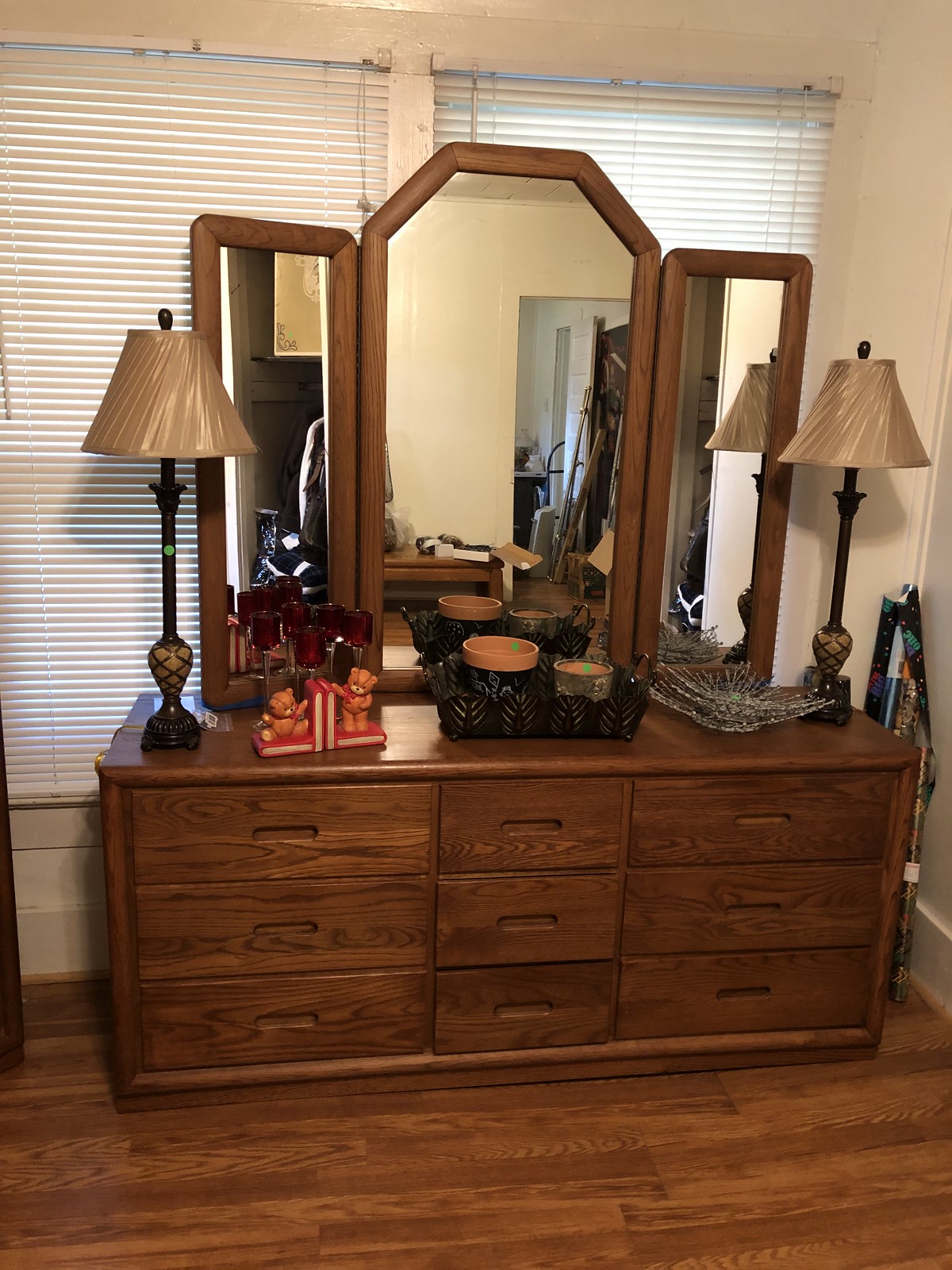This image captures a detailed view of a cozy bedroom featuring a distinctive wooden dresser, which boasts a medium brown stain that matches the hardwood floor. The dresser is positioned below two side-by-side windows with closed white mini blinds that allow a slight trickle of light to enter the room. The walls are painted off-white, adding to the serene ambiance.

The dresser itself is quite unique, equipped with nine drawers arranged in three columns and three rows. The outer columns host larger drawers, while the central column consists of narrower drawers, each equipped with a slit handle reminiscent of a 1970s design. Mounted atop the dresser is an elegant trifold mirror. The central section of the mirror has an angled or hexagonal shape that nearly reaches the top of the windows, flanked by two rectangular, wood-framed mirrors that fold out on either side.

Adorning the dresser are several decorative items: two matching table lamps with plastic-wrapped tan shades resembling candlestick-style bases, positioned symmetrically on either end. Between the lamps, a pair of charming care bear bookends cradle a couple of books. Additionally, a metal tray holds terracotta bowls or planters without any plants, and a low crystal bowl adds a touch of glass elegance. In the room’s corner, behind the dresser, a rolled-up poster can be seen lying against the wall, completing the scene with a casual touch.